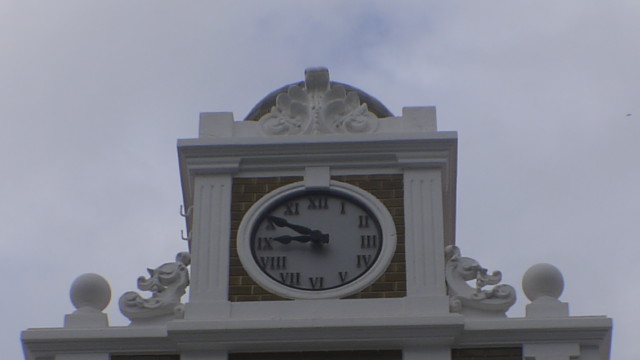This photograph captures the facade of an ornate building, likely European in the Rococo style, focusing on an intricately designed clock tower. The clock features a white face with black Roman numerals from 1 to 12, and has black hour and minute hands. It is set against a red brick background, surrounded by an elaborate white molding that forms a square outline. The clock is integrated into an ornate part of the building, which includes symmetrical white pillars on either side. At the top of these pillars, there are matching plinths adorned with statues, including a man's head resembling a gorgon's head at the apex, and other L-shaped and reverse L-shaped sculptures that appear to portray humans, accompanied by two globes resting on rectangular blocks. The sky above is mostly overcast with lots of white clouds, allowing just a hint of blue to peek through.